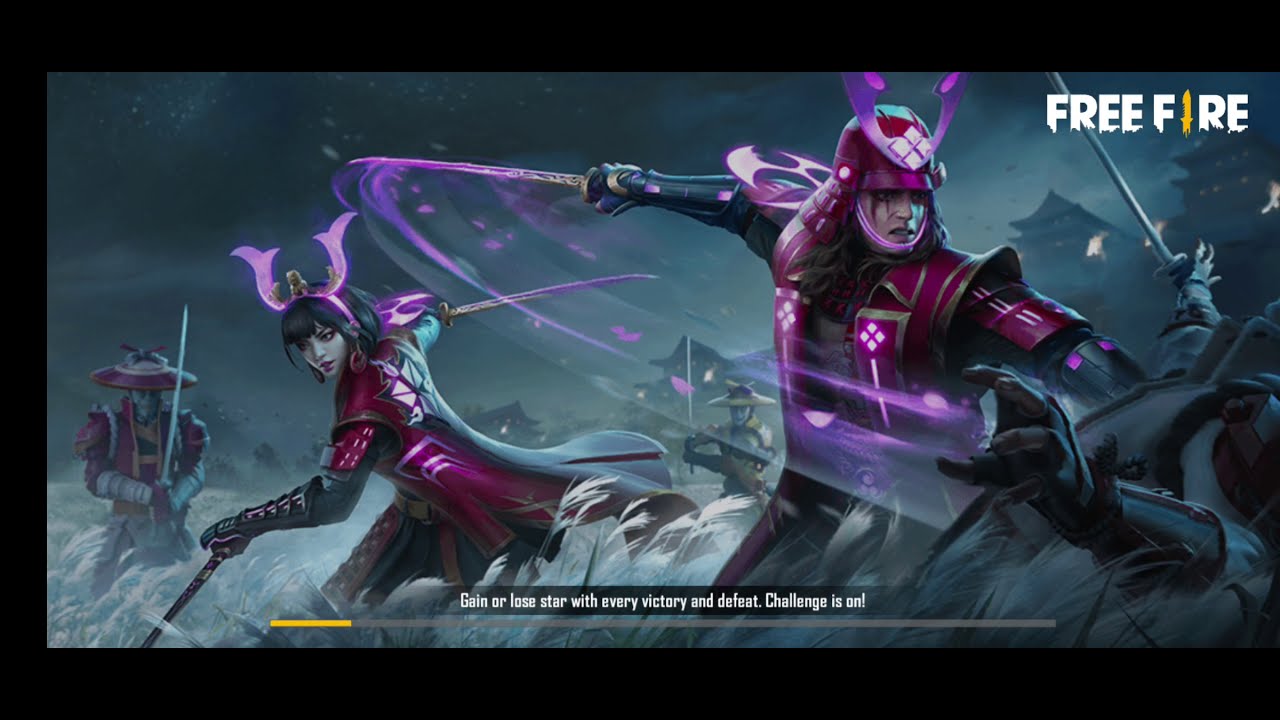The horizontal rectangular image appears to be a loading screen from a video game, featuring vibrant and detailed artwork. The image is bordered by black on the top left and bottom, while the right side remains borderless. At the center-right, a prominent female warrior, donned in purple samurai armor with a purple helmet and black gloves, strikes a dynamic pose wielding a pole in her left hand and a glowing energy sword in her right. Beside her, another female soldier similarly dressed in samurai armor emanates a purple hue from her weapons, emphasizing the intense action scene.

In the background, albeit blurred, traditional Japanese houses are faintly visible, contributing to the setting's authentic aesthetic. A menacing figure, possibly an antagonist, clad in distinct samurai attire with a circular helmet, stands poised for battle on the far left side of the image. The overall color palette melds vivid purples and yellows with somber grays and blacks, suggesting a nighttime scenario illuminated by subtle highlights.

The top right corner bears the game's logo, "Free Fire," where the 'I' uniquely transforms into a golden sword. Below, white text reads, "Gain or lose STAR with every victory and defeat. Challenge is on." Further below, a loading bar, partially filled at around 10-15% and shaded yellow, hints at the game's progression status, contrasting against the dark backdrop.